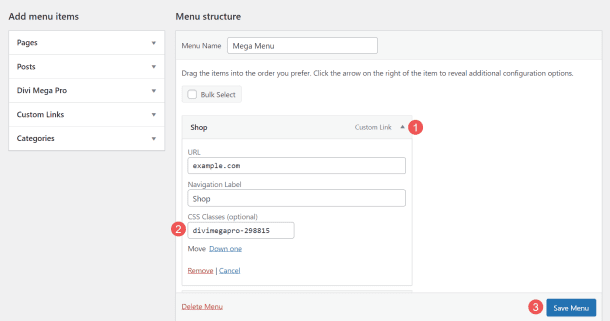The image displays a webpage interface for customizing a website menu. At the top of the page, there is a heading titled "Add Menu Items" with a drop-down menu featuring various options such as "Pages," "Posts," "dbMegaPro," "Custom Links," and "Categories," each accompanied by grey drop-down arrows.

Below this, there is a section labeled "Menu Structure," where users can set the "Menu Name," which in this case is "MegaMenu." The section instructs users to drag the items into their desired order and to click on the right-hand arrow of each item to access additional configuration options.

A "Bulk Select" box is available for multiple selections. Below this, there are specific menu items listed. The first item is titled "Shop," identified as a custom link with a red badge displaying the number "1." It includes fields for "URL" (filled with "example.com") and "Navigation Label" (filled with "Shop"). Optional CSS classes can be added here.

Another item, "DivineGopPro," is marked with a red badge showing the number "2" and includes a unique identifier "298815."

At the bottom of these options, there are several buttons including a "Move" button, a light blue "Down 1" button, a red "Remove" button, a blue "Cancel" button, and a red "Delete Menu" option. At the very end, a light blue button labeled "Save Menu" is available for saving the menu settings.

The majority of the page features a grey and white background with black text for greater readability.